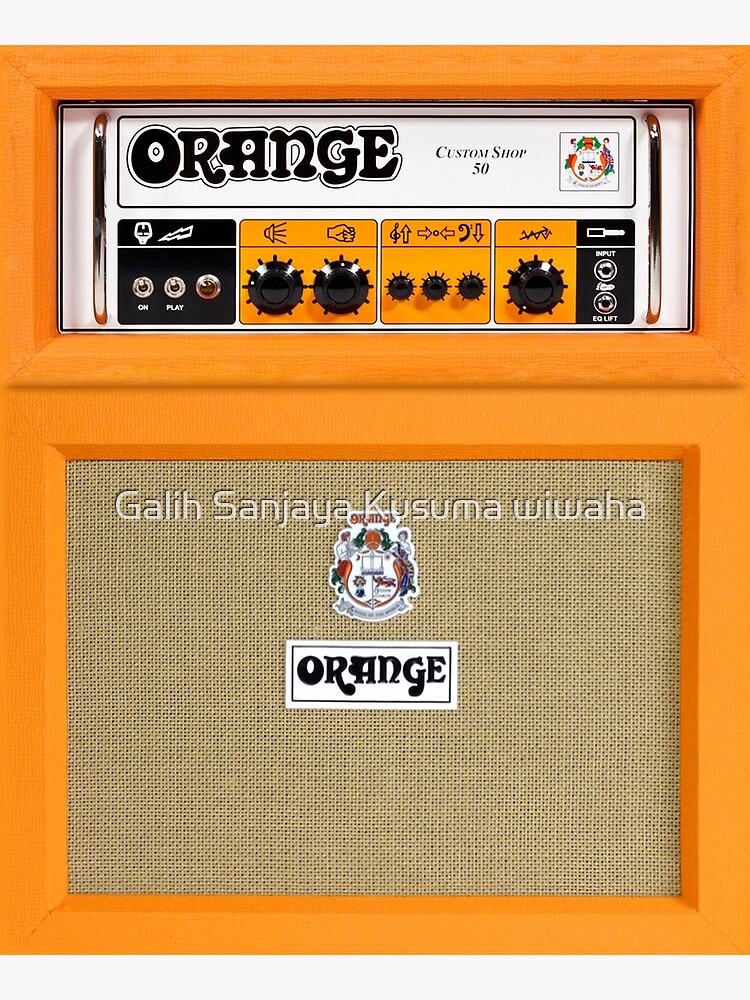The image depicts a bright orange, box-shaped audio equipment, potentially for a guitar or musical instrument, featuring various control elements. The top portion prominently displays "Orange" in large, bold black letters, followed by "Custom Shop 50" to the right. The equipment has a mesh material on the front bottom portion, also containing the "Orange" logo and the name "Kusumawiwaha" just above the logo. The piece includes several dials and knobs for adjusting volume, changing channels, and modifying pitch, as well as buttons labeled "on" and "play." There are also input and output areas for connecting cables, indicating its versatile functionality. Additionally, two metallic handles flank the sides, and the item is further adorned with an emblem or seal on the upper right side, emphasizing its distinct design and branding.